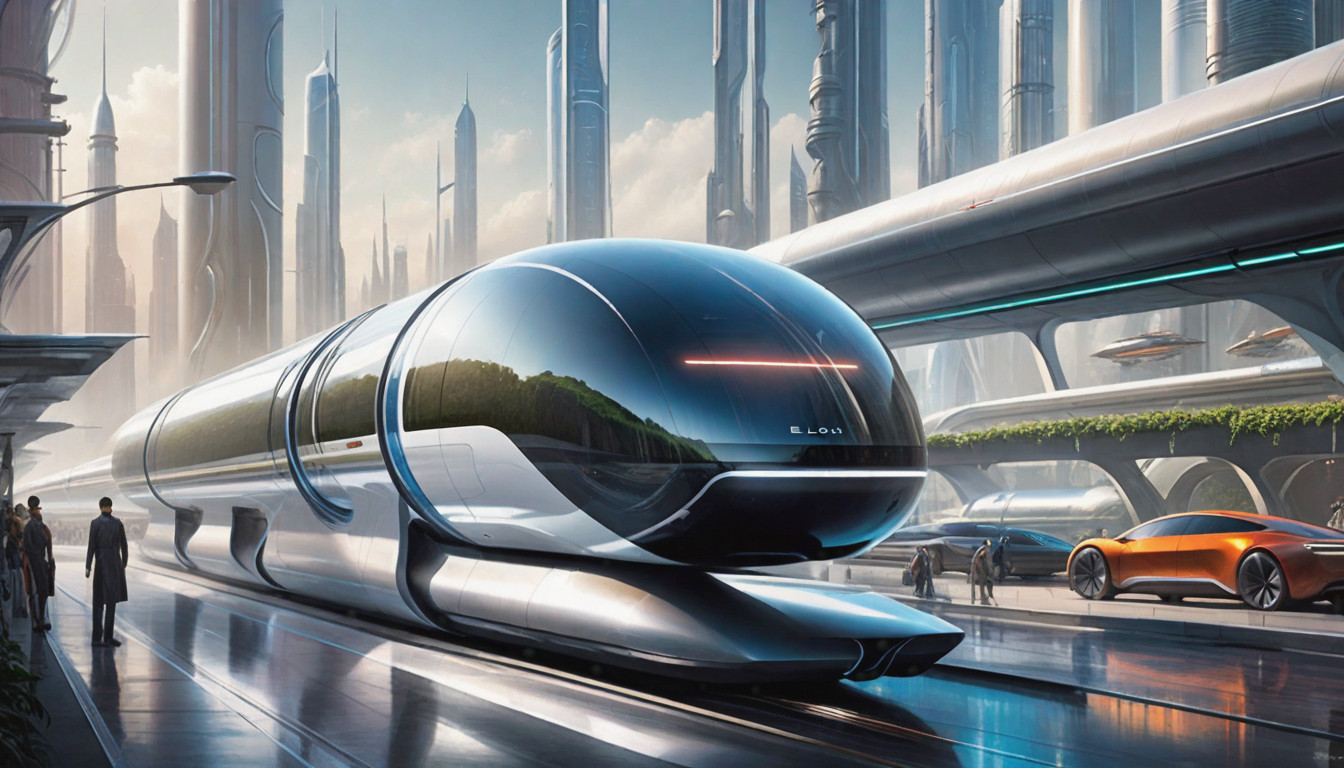This image features an AI-generated illustration of a highly advanced, futuristic setting. Dominating the scene is an ultra-modern, sleek train, resembling a supersonic tube with an entirely glass upper section and a polished silver reflective lower half. The train is seen whizzing by, drawing attention to its innovative design and the non-traditional embedded tracks on a polished paver and concrete floor. 

On the far left, a few people stand close to the train, likely passengers. To the other side, near the train, there are a couple of futuristic cars—one in a striking bright orange color and the other in a grayish hue. 

Above, the sky is dotted with a few flying vehicles, adding to the advanced atmosphere of the illustration. Towering in the background are massive skyscrapers, far taller and more architecturally ambitious than those seen in contemporary cities, some boasting spires that ascend dramatically into the sky. This elaborate cityscape underscores the overall theme of extreme futurism and innovation.